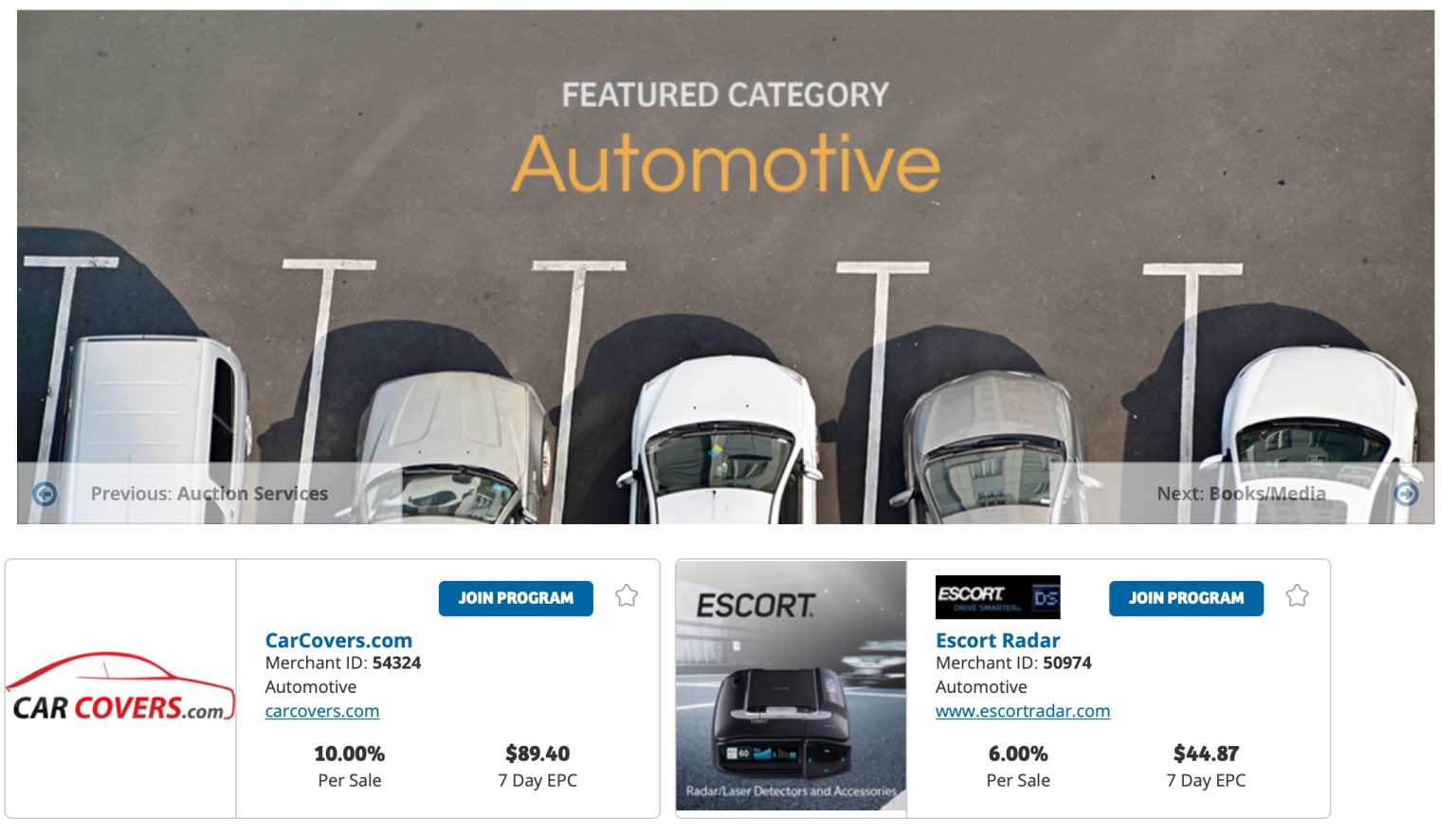On an e-commerce website specializing in car covers and automotive accessories, a striking image occupies half of the webpage. The photograph showcases five white vehicles evenly spaced in a parking lot, delineated by stark white lines. The fleet of cars consists mostly of sedans, with the exception of a white van positioned on the far left. Towering text overlays the image, declaring "Featured Category" in white, while "Automotive" is emblazoned in bold, orange letters. 

In the bottom-left corner of the image, a small box indicates "Previous Auction Services." Directly beneath the main picture, two detailed boxes provide further information:

1. The first box highlights CarCovers.com with the brand name split into contrasting hues—'car' in black and 'covers' in red. It includes the merchant ID "54324 Automotive" and repeats the CarCovers.com URL twice, once underlined and once plain, both in blue. Additional details note a 10% commission per sale and a 7-day EPC (Earnings Per Click) of $89.40. A blue "Join Program" button, accompanied by a star, encourages engagement with the program.

2. The second box features a photo of an Escort Radar, a radar and laser detector designed for automotive use. This box lists the merchant ID as "50974 Automotive" alongside the website information, promising a 6% commission per sale and a 7-day EPC of $44.87. It similarly includes a blue "Join Program" button next to a star.

Together, these elements create a comprehensive and appealing showcase for the automotive products and affiliate opportunities available on the site.